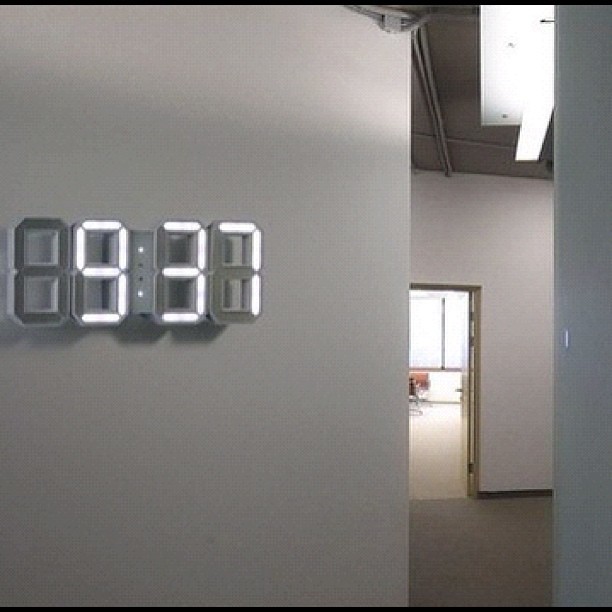The image depicts what appears to be the interior of an office building or possibly a home, characterized by a light gray, possibly tiled ceiling with long fluorescent lighting fixtures. Dominating the left side of the scene, a prominent digital clock is mounted on the wall, featuring large, bright white seven-segment numerals that read "937". The clock's design emphasizes its digital nature, with numbers appearing in the segmented form found in traditional digital clocks without additional embellishments. The wall itself is a plain light gray, extending across much of the image. Toward the right, there is an open doorway leading to another room. Inside this adjoining space, a reddish chair is faintly visible, positioned in front of a large window that does not reveal anything outside. The overall composition of the image creates a minimalist yet slightly industrial ambiance.